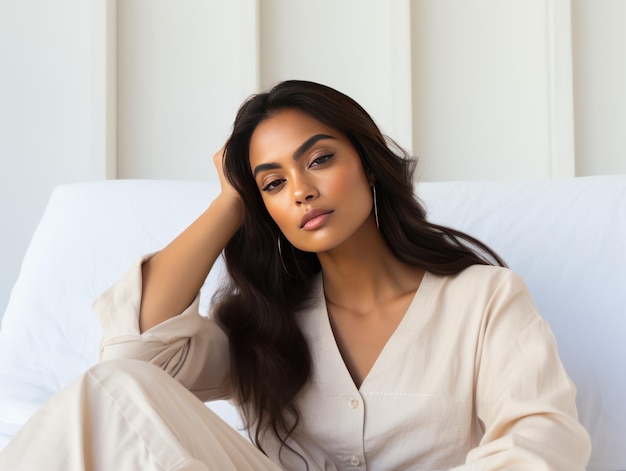In this bright, airbrushed photo, a beautiful woman with olive skin and long dark hair, possibly an Indian model, is seated alone in a bed adorned with white linens against an off-white wall. She is wearing an off-white pajama set with buttons, possibly in a very light pink hue, and has one leg elevated while resting her head on her right arm to the left side of the image. Her makeup is meticulously applied, featuring a lot of contouring, and she is accessorized with earrings that accentuate her collarbones and the slenderness of her neck. With her eyes partially closed, she conveys a sense of tiredness or readiness for romantic activities. The background behind her shows some vertical lines, adding a subtle texture to the otherwise serene, well-lit setting.